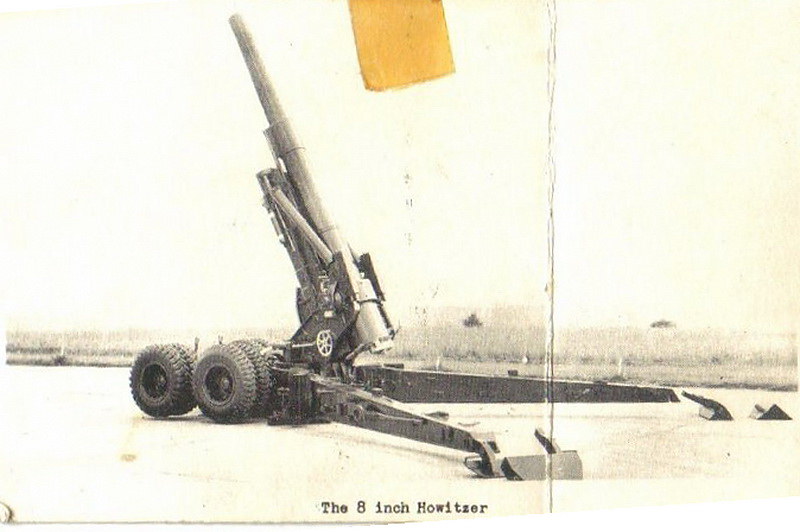This is a vintage black and white photograph, likely from an era gone by, depicting an 8-inch howitzer. The image, which has been folded, shows a prominent crease running vertically about two-thirds of the way across. A piece of old cellophane tape, now a yellowed orange with age, is adhered to the top center, suggesting it was once displayed on a wall. The photograph is rectangular and landscape in orientation, exhibiting signs of wear with a faded, slightly beige tint.

The subject of the photograph is the large howitzer, mounted on a metal frame with bracing arms pointing to the right. It rests on a set of large wheels, with at least four visible on one side. The central component of the howitzer, the barrel or "cannon tube," is positioned upward and slightly to the left. The background is heavily grayed out, making the horizon line and landscape barely discernible. Below the howitzer, along the bottom margin, is a typewritten label that reads "the 8 inch howitzer." The entire scene is captured in a classic vintage photography style, evoking a sense of historical significance.